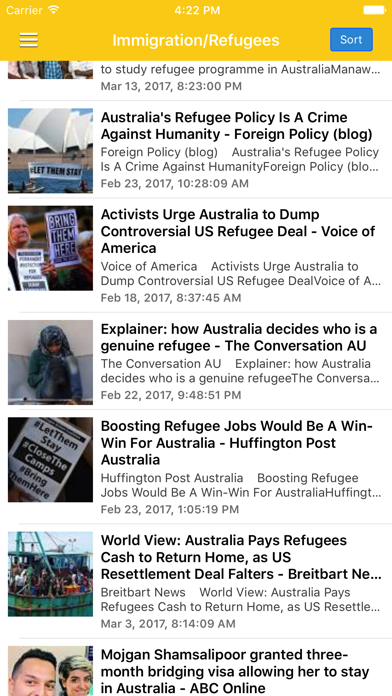Header bar: At the top of the page, there is a blue "Sort" button on the right and the text "Immigration & Refugees" on the left. Above this section, the page displays the number "422" in bold. To the left of the "422," there are three horizontal white lines. This entire section is encased in an orange header bar.

Article: Below the header, an article starts, focusing on Australia's refugee program. The introductory part of the article is not visible. 

To the left of the article, there is an image dated March 13, 2017. Underneath the image, the text reads, "Australia's refugee policy is a crime against humanity." This appears to be a segment from a blog titled "Foreign Policy Blog," with the same headline, "Australia's refugee policy is a crime against humanity," dated February 23. The accompanying image is of the Sydney Opera House.

Another photograph shows an elderly lady protesting, holding up pictures. One of the pictures she holds has the text "Bring them here," urging Australia to abandon a controversial U.S. refugee deal. This image is credited to "The Voice of America," dated February 18.

A section titled "Explainer: How Australia Decides Who is a Genuine Refugee" from "The Conversation AU" is dated February 22.

Another segment titled "Boosting Refugee Jobs" includes a hashtag "#LetThemStay" and slogans like "Close the Camps," shown on a flyer held by someone. 

An image of a shipping boat is captioned "World View: Australia Pays Refugees Cash to Return Home."

Lastly, there is a mention of Morgan Shams Lapoor being granted a three-month bridging visa that allowed her to stay in Australia, with a reference to ABC Online.